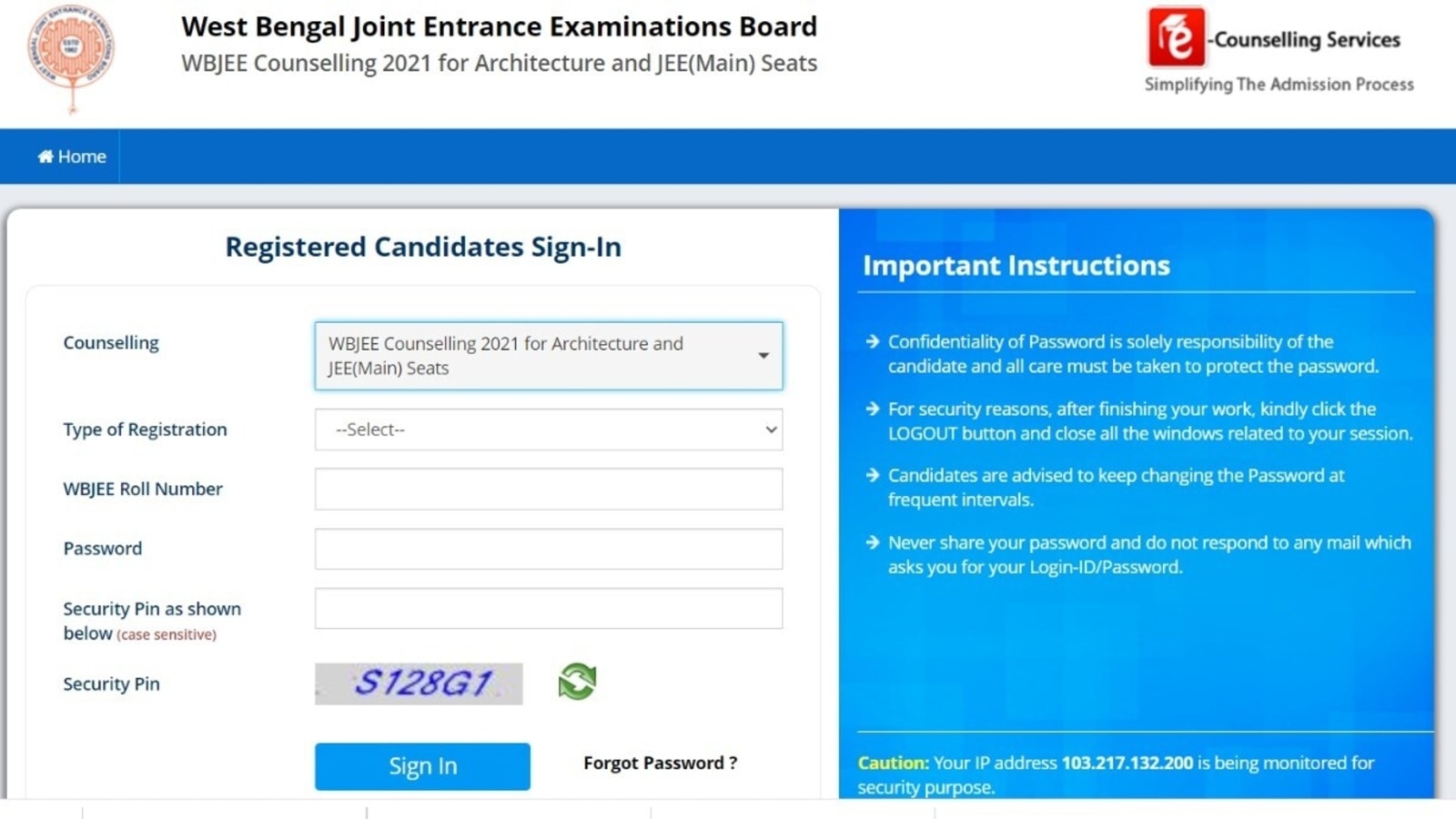The image depicts the log-in page for the West Bengal Joint Entrance Examination Board (WBJEE) Counseling 2021 for Architecture and JEE Main Seats. At the top of the page, there is a blue navigation bar with a home icon and the label "Home." Above this bar, the page header reads, "West Bengal Joint Entrance Examination Board, WBJEE Counseling 2021 for Architecture and JEE Main Seats."

Below the header is a section labeled "Counseling." This section reiterates "WBJEE Counseling 2021 for Architecture and JEE Main Seats" and features a drop-down arrow for selecting the type of registration. 

The form fields that need to be filled in include:
- "WBJEE Roll Number" (which is currently blank),
- "Password" (which is also blank),
- A "Security Pin" field, highlighted in red text indicating that it is case sensitive and currently blank. 

Displayed below the field for the security pin is a gray box containing a blue text code "S128G1" with a refresh icon of green arrows next to it, allowing for the generation of a new security pin.

Finally, at the bottom of the section, there is a blue "Sign In" button followed by a "Forgot Password?" link indicated by a question mark. The left side of the page summarizes the required fields: "counseling type of registration, WBJEE Roll Number, Password, Security Pin," suggesting that users must complete these fields to proceed.